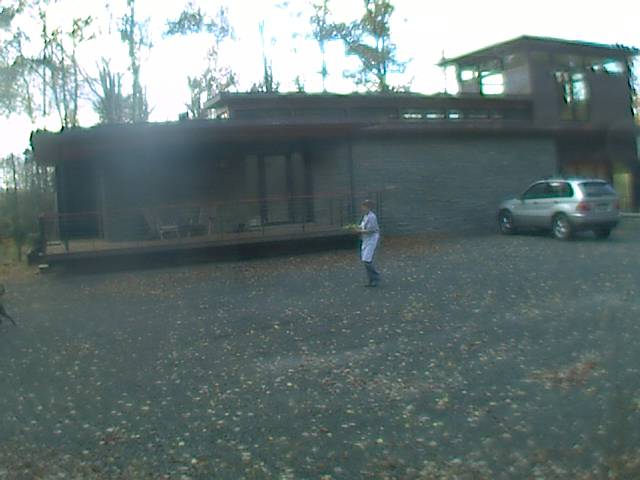This outdoor image depicts a modern, multi-story residential building with a layered design. The building features a front deck with a porch that includes two chairs on the left of the entrance, and a railing. To the right of the entrance, there's what appears to be a gray wall, potentially a garage, with a silver, compact SUV parked in front of it. The house spans several levels, with multiple windows indicating a wide view of the surrounding area. In the foreground, on the black asphalt street, yellow leaves and petals are scattered, suggesting it's fall. A person, whose details are unclear but who might be wearing an apron or dress, is walking towards the left, carrying what seems to be a tray of something. The background is filled with large, thin trees showcasing their leaves, and the lighting suggests it is a sunny or slightly overcast day.